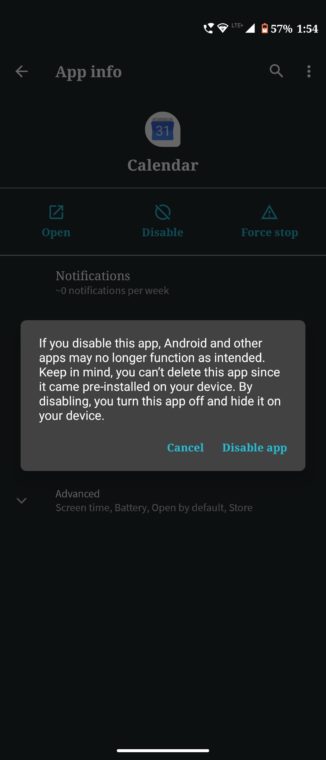A detailed screenshot depiction shows a smartphone display with a pop-up box prominently overlaying a dark screen. Indicators at the top of the screen include a phone icon, a Wi-Fi symbol, and a battery icon displaying 57% charge. Positioned to the left is a timestamp denoting 1:54. 

Below the status bar, a title row showcases a left-facing arrow labeled "Back," following by "App Info." To the right of this, there are search and three-vertical-dot icons for additional options. Centered below these icons is a calendar icon, marked with the number "31" and labeled "Calendar."

This section is followed by three interactive tabs: "Open" on the left, "Disable" in the center, and "Force Stop" on the right. Beneath these options, a notification indicator shows "Zero notifications per week."

Dominating the upper part of the screen, a gray pop-up box with white text warns: "If you disable this app, Android and other apps may no longer function as intended. Keep in mind, you can’t delete this app since it came pre-installed on your device. By disabling, you turn this app off and hide it on your device." It provides two selectable options at the bottom: "Cancel" and "Disable App."

Further below, a drop-down arrow reveals additional options related to "Advanced," "Screen Time," "Battery," "Open by Default," and "Share." Capping the display, a thin white line at the bottom represents the Home button.